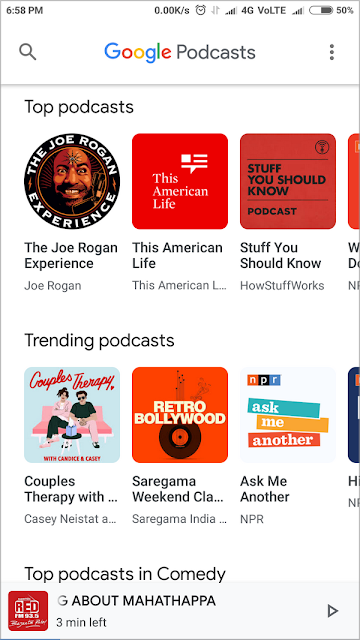A detailed screenshot of the Google Podcasts app captured on a smartphone is shown. The time displayed in the upper left corner of the phone is 6:58 PM, and the battery life is at 50%. The device is connected to the 4G LTE network as indicated by the status icons at the top of the screen. Below these indicators is the Google Podcasts interface, highlighted by the Google logo in its signature multicolored letters followed by the word "Podcasts". On the right side of this bar is a magnifying glass icon (suggesting a search feature), and to the left are three vertical dots (likely indicating additional options or settings).

The main part of the screen displays a section titled "Top Podcasts". The first podcast listed is "The Joe Rogan Experience" by Joe Rogan. Following this is "This American Life" and alongside it, "Stuff You Should Know". However, only three of these top podcasts are fully visible, with the fourth one partly cut off due to the screen size.

Beneath this section, there is a "Trending Podcasts" category. Within this section, several podcast titles are partially visible. Notable entries include "Couples Therapy with…", which is cut off, "Sarah Game Weekend Castles", and "Ask Me Another". The text "Ask Me Another" appears again in a further listing, suggesting it might be a recurring feature or category.

Overall, the image effectively captures the layout and some specific features of the Google Podcasts app interface, providing insight into the user's current connectivity and battery status on their smartphone.